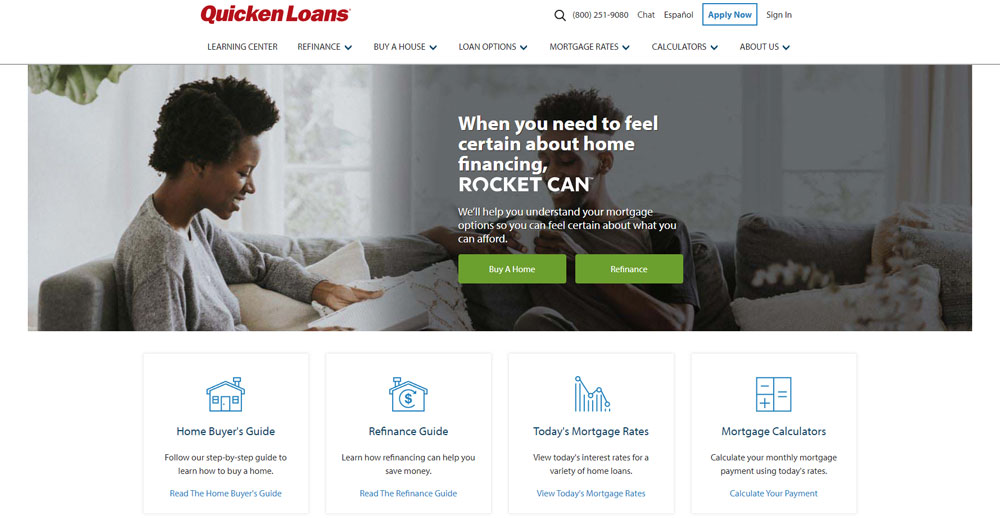**Detailed Caption:**
 
The top portion of the image features a white background. In the left-hand corner, there’s red text that reads "Quicken Loans." Adjacent to this, on the right-hand side, is a black magnifying glass icon. Next to the magnifying glass, it says "(800)" followed by the phone number "232-5190". Below this information, there is text indicating "Chat Español," suggesting the availability of Spanish-speaking customer support. 

A blue outline box appears in the middle section. Within this box, against a similarly colored background, blue text prompts "Apply Now." Below this, in black text, there's an option to "Sign In." On the left side, menu options in black text read: "Learning Center," "Refinance," "Buy a House," "Loan Options," "More Coverage," "Calculators," and "About Us." A black line runs horizontally across the section beneath these options.

The lower part of the image features a living room scene with a woman and a man sitting on a couch. The woman, situated on the left, has an Afro hairstyle adorned with a headband and is wearing a gray shirt while engrossed in reading a book. On the right, the man appears to be either her husband or partner; his Afro hairstyle suggests a possible time period. He is wearing either a black or gray shirt (it's indistinct due to blurriness in that area) and holding a teacup. Overlayed on his face in white text is the message: "What you need to feel certain about home finance. Rocket can help you understand your mortgage options so you can feel certain about what you can afford."

At the bottom, there are two green boxes. The first box, in white text, says "Buy a Home," and the second box says "Refinance." Below these, a header reads "Homeowner's Guide" followed by a link to the "Refinance Guide" and "Today's Mortgage Rates" in blue text.